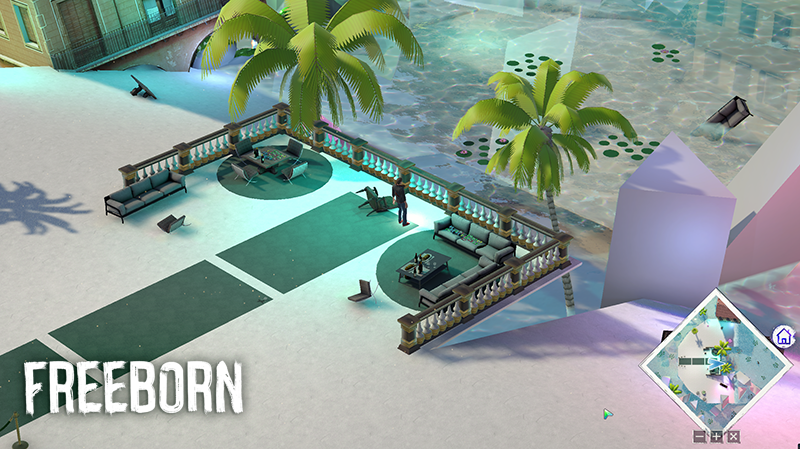The image is a digital art graphic, likely a screenshot from a video game titled "Freeborn," as indicated in the lower left corner. The scene is set at a beach or a swimming pool environment, featuring a large patio area elevated above or next to the water. This seating area is surrounded by a stone railing forming an elongated U-shape, and it has multiple green seating sections, including green couches and chairs. There is also a person standing among the overturned chairs. Leading to this area is a walkway adorned with three pieces of green carpet.

Two tall palm trees stand at each corner of the seating area, casting shadows on the concrete-like white floor. On the right side, just beside the rightmost palm tree, there's a prominent purple triangular column. Additionally, a brown building is visible in the background, in the top left corner. Notably, there is a sofa floating in the water, which could be a pool or part of the ocean. In the bottom right corner of the image, a minimap provides a visual aid of the surrounding section within the game.